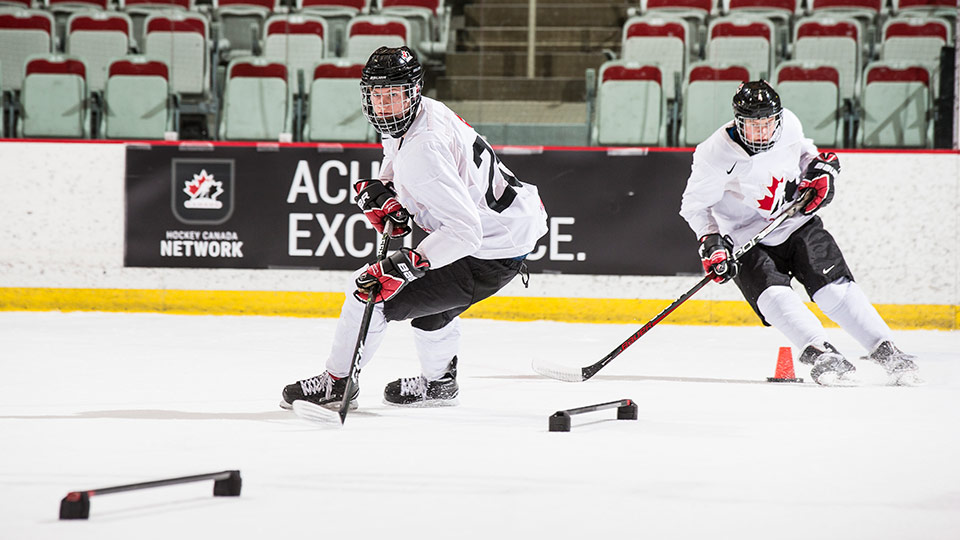The image depicts a professional-style indoor ice hockey practice session featuring two junior male hockey players wearing full-face shields on their black helmets. They are dressed in white Team Canada jerseys adorned with a red and black Maple Leaf logo and black numbers, complemented by black pants, white socks, black skates, and black and red Bauer-branded hockey gloves. The player on the right is seen holding a Bauer stick, while the player on the left uses a CCM stick. Both players are navigating through a skating drill around an orange pylon and other stick-handling training tools suctioned to the ice. The background showcases a black banner with partial visible text, "Hockey Canada Network" alongside a red, white, and black Maple Leaf logo. The rink's ice is bordered by white and yellow lines, and the empty stands feature red and light-colored seating.